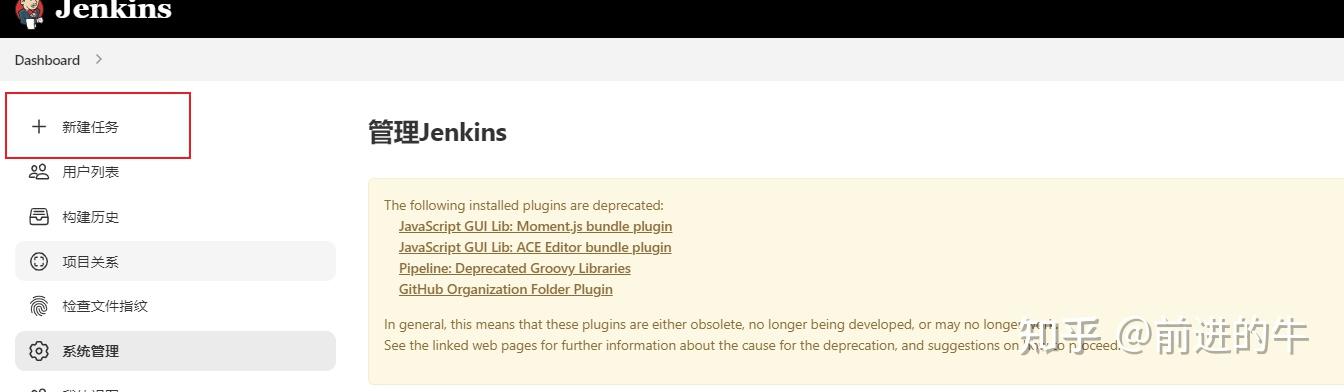A screenshot of the Jenkins Dashboard interface is displayed prominently. Jenkins, stylized as "J-E-N-K-I-N-S," is represented by a graphic of a well-dressed gentleman in a blue suit and red bow tie, holding a white coffee cup. The character sports a mustache and is placed above a header labeled "Dashboard," which features a red arrow indicating additional information is available.

The interface displays various elements primarily adorned with Asian script. The first box, located at the top left, includes a plus sign and is filled with Asian characters. Below it, there are two options for adding usernames, each accompanied by Asian text. Additional icons include a file folder with Asian writing, a circle with directional arrows, another section with Asian text specifying fingerprint settings, and a settings icon. To the right, the word "Jenkins" is displayed, also surrounded by Asian characters.

In English, a yellow notification box alerts users that several installed plugins are deprecated. They include JavaScript GUI Library, Moment.js bundle, Ace editor, Pipeline Deprecated Groovy Library, and a GitHub-related plugin. It is noted that these plugins are either obsolete or no longer actively developed. The notification advises users to visit the linked webpage for more details about the deprecation causes and suggestions for moving forward.

At the top of the page, a white header bar spans the entire width of the website, while a black horizontal bar extends similarly beneath it. The interface provides a comprehensive view of Jenkins' functionalities and essential updates with visual and textual information.